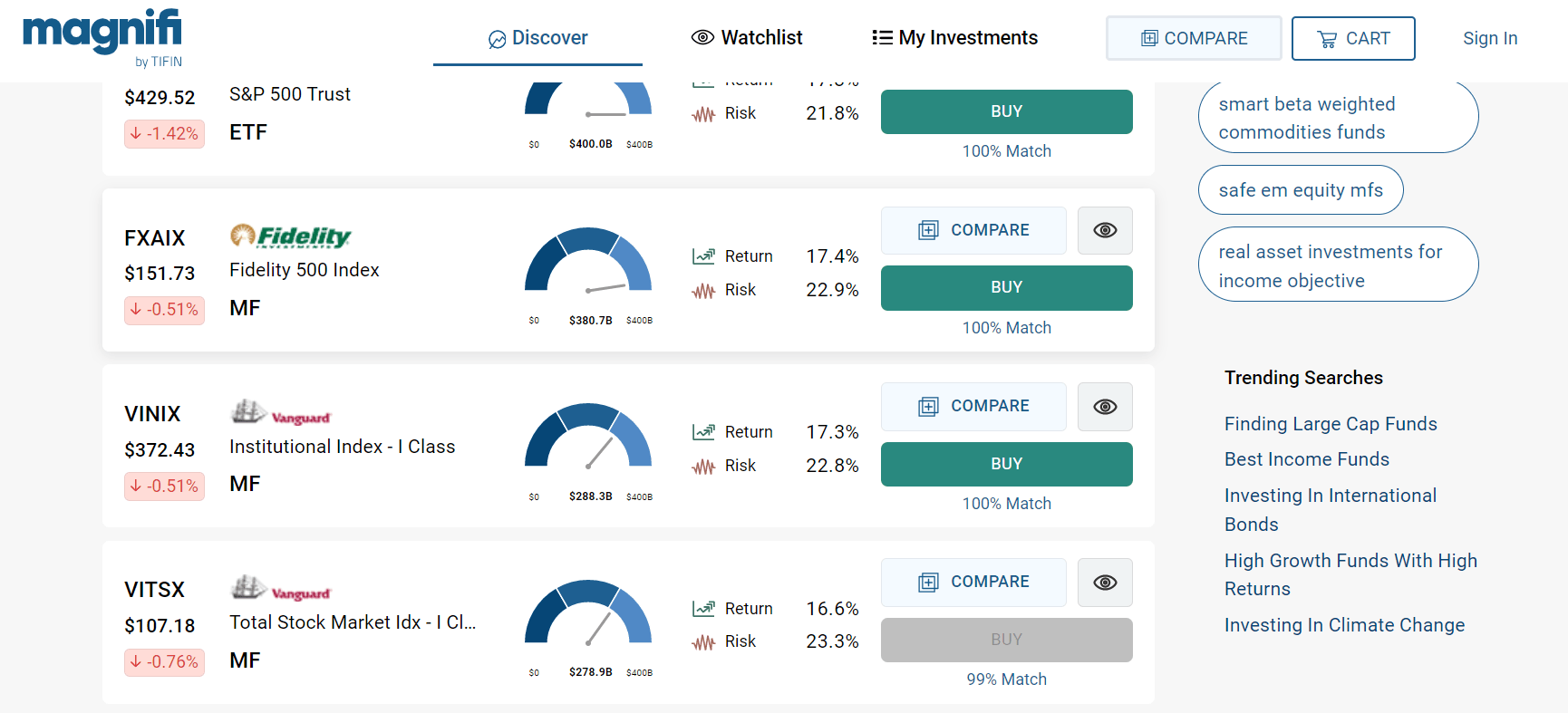This cropped screenshot captures a view of the Magnify by Tiffin website. At the top left corner, there is a logo that says "Magnify by Tiffin." Adjacent to the logo on the right, the navigation bar features options such as Discover, Watchlist, My Investments, Compare, Cart, and Sign In, with Discover being selected and highlighted by a blue bar beneath it. The main section of the page contains a vertically aligned series of white boxes, each representing different holdings, and the page is scrolled down to its bottom.

Visible at the very top of the screenshot is the bottom of a box, just above a detailed section for Fidelity. This particular box displays the stock name FXAIX on the left side, with its current price beneath it and a red box indicating a price drop. Centrally located within the box is a dial featuring three blue segments (dark blue, medium blue, and light blue) with the dial positioned all the way to the right. Additionally, there are labeled metrics for return and risk with associated percentages, and options to Compare, represented by an eye icon, and Buy on the far right. The box also notes a "100% match" in small blue letters.

The two subsequent boxes are visible, following the same layout: the first for Vanguard Institutional Index, and the next for Vanguard Total Stock Market Index. 

On the right side of the screenshot, a gray panel presents a series of informational topics within rounded bubbles. The topics include "Smart Beta Weighted Commodities Fund" at the top, followed by "Safe M Quality MFs," and "Real Asset Investments for Income Objective." Below these topics, the panel lists "Trending Searches" in small black font, accompanied by a set of current trending search topics.